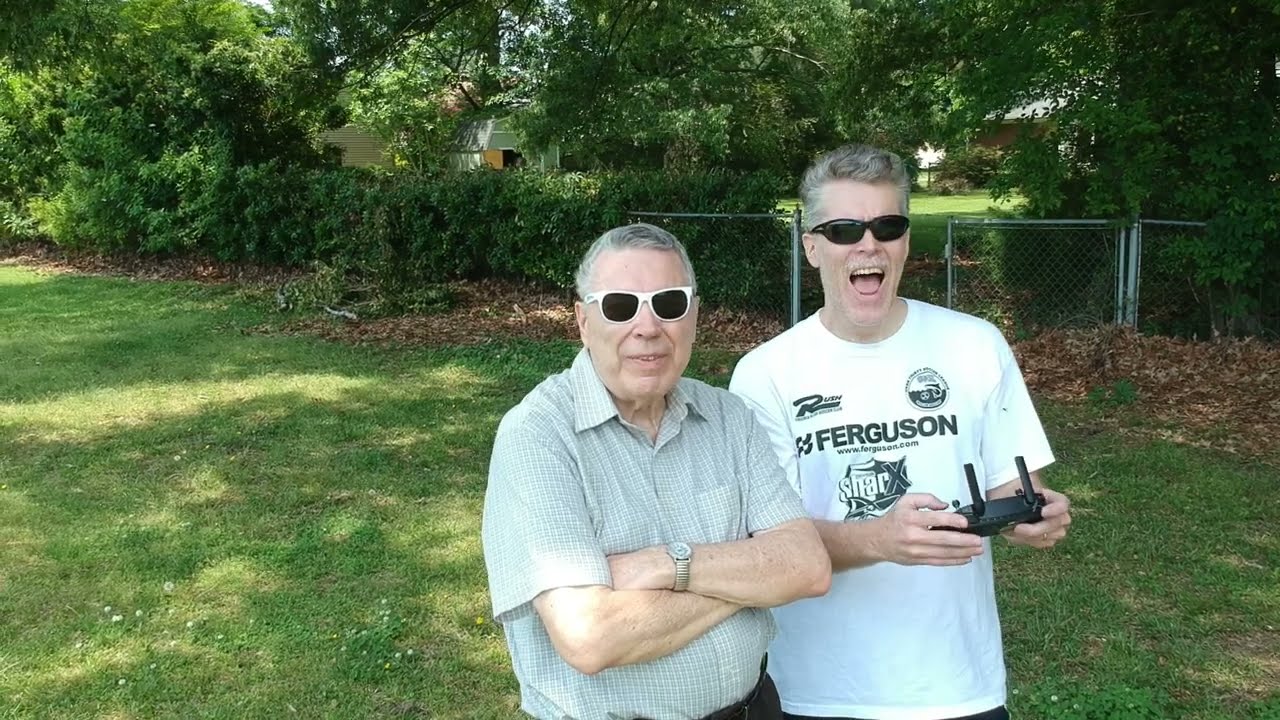This is a vibrant photograph of two older men standing in a spacious backyard that features lush greenery, including a green lawn, dense bushes, and tall trees, with a wire fence in the background and a couple of houses partially visible through the trees. The man on the left appears to be around his 60s or 70s, with white hair, white sunglasses, and wearing a light-colored, long-sleeve shirt. He has his arms crossed in front of him. To his right, but our left, stands a slightly younger man, probably in his mid-40s, wearing black sunglasses and a white t-shirt with "Ferguson" printed on it. His mouth is open in a hearty laugh, revealing his teeth and tongue as he holds a joystick, likely used to control the drone capturing this eye-level shot. Both men are radiating joy and camaraderie, perfectly framed in their idyllic backyard setting.